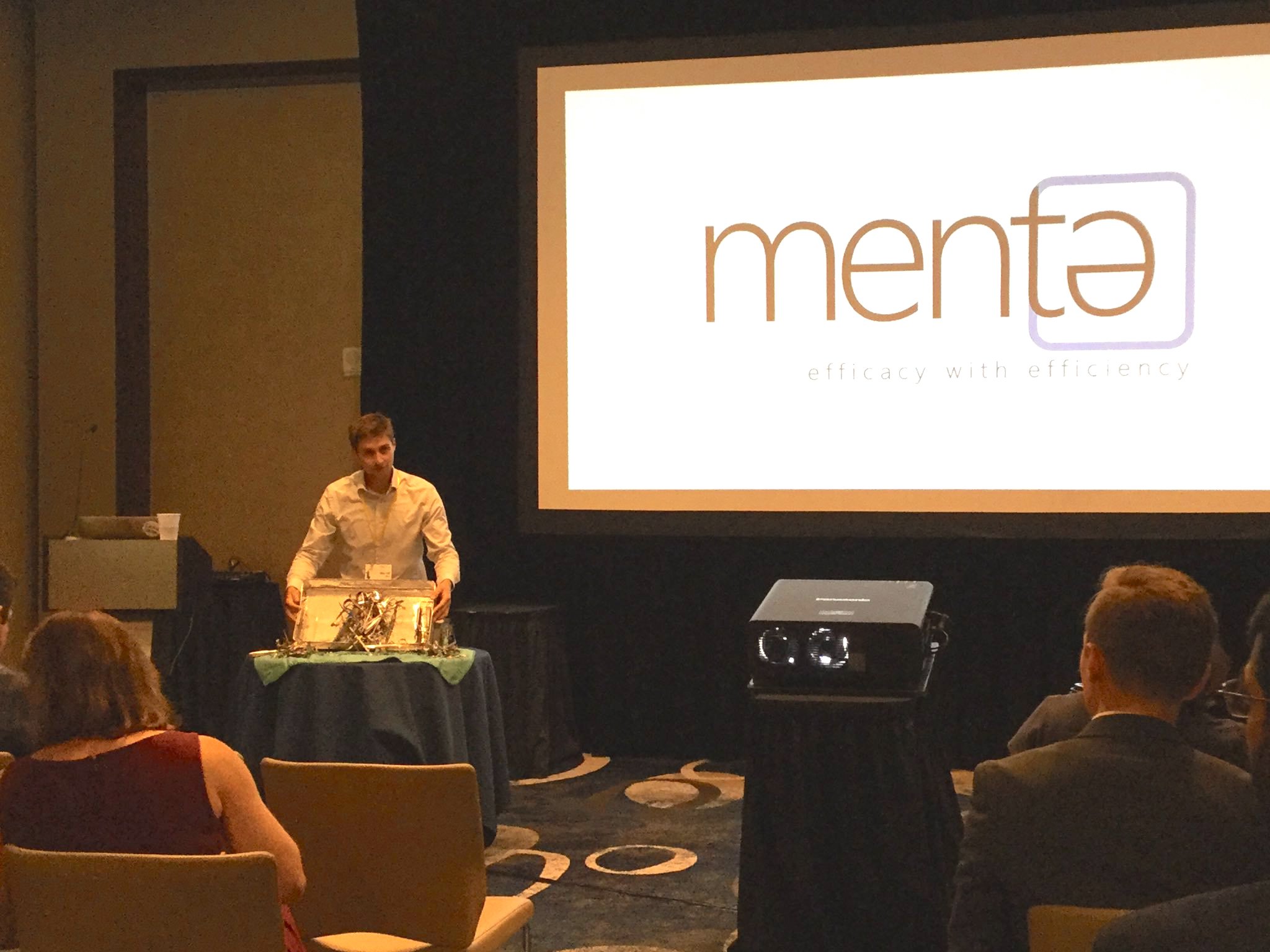In this landscape-oriented image, we see a meeting taking place inside a room. Central to the image, a man in a long-sleeved white or white-tan buttoned-up shirt is standing at the front, engaging with the audience. He is holding a platter or display object over a table that features both a blue tablecloth and a smaller green tablecloth. The table is round and neatly covered.

Behind the man is a projection screen, bordered in orange, displaying the text "M-E-N-T-E," with the final "E" upside down and both the "T" and "E" encapsulated in a roughly square, purplish-gray box. Directly below this text is a smaller caption that reads "Efficiency VIF Efficiency" or "Efficacy with Efficiency" – the latter part being hard to discern. To the left of the projection screen, there's a podium equipped with a microphone and a black cover draping part of the background, as well as a glimpse of the room’s wall.

The audience, seated on hardback, almost orange-colored chairs, is captured with their backs to the viewer. Some attendees are dressed formally, with a couple of men in suits and ties, and a woman in a dress visible in the aisle rows. In the middle of the room, a projector positioned on a stand is casting the image onto the screen. The overall atmosphere and attire suggest a somewhat formal, perhaps slightly dated setting.